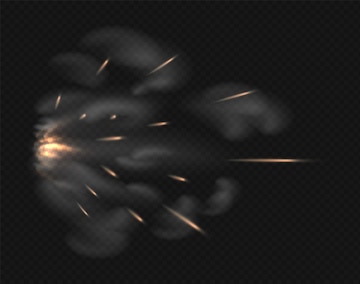The image depicts a dynamic explosion-like effect against a predominantly dark background, which has a subtle checkerboard pattern of gray and black squares. At the far left, three primary flames can be distinguished: a large central flame flanked by two smaller ones that angle upward and downward. From this ignition point, a dense smoke cloud billows to the right, featuring various shades of gray. Within the smoke, vivid streaks of reddish-orange light shoot out, becoming paler and more diffuse as they extend away from the source. These streaks vary in length, with those closer to the origin being shorter and more numerous, gradually elongating and spreading out as they move across the image. The overall visual effect suggests the momentary burst of sparks and smoke one might see if capturing a gunshot precisely at the moment of firing, but with the gun itself removed, leaving only the fiery aftermath and drifting smoke.